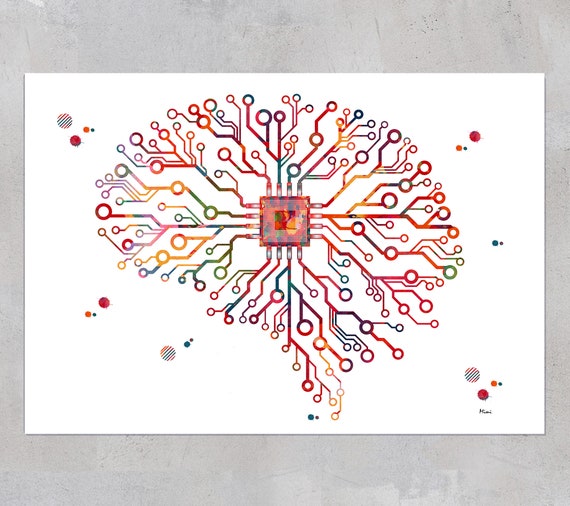The image portrays a landscape orientation with a refined, creamy marble backdrop featuring shades of gray interspersed with light cream accents. Against this backdrop, a white rectangle serves as the canvas for the central digital artwork. At the core of this arrangement lies a transparent red square, bordered by a more intense red outline. Radiating from this red square, a multitude of colorful lines—ranging from red, orange, and yellow to green, blue, and purple—extend outward, each terminating in colored circles representing diverse hues.

The overall composition bears a resemblance to a brain silhouette, reminiscent of synaptic connections or a circuit board. The lines branching from the central red square evoke the intricate paths of neural or electrical connections, akin to a network or train map. The organized chaos of the colors and lines suggests various nodal points or stops. 

Amidst this colorful web, distinct clusters of dots are situated in specific areas: three dots (light blue and red) ascend toward the left-hand side, while two red dots move toward the right-hand side. The bottom right-hand corner showcases around four dots in light green and red, contrasting with the completely white bottom left corner. Overall, the piece masterfully blends artistic and conceptual elements, evoking both biological and technological themes.